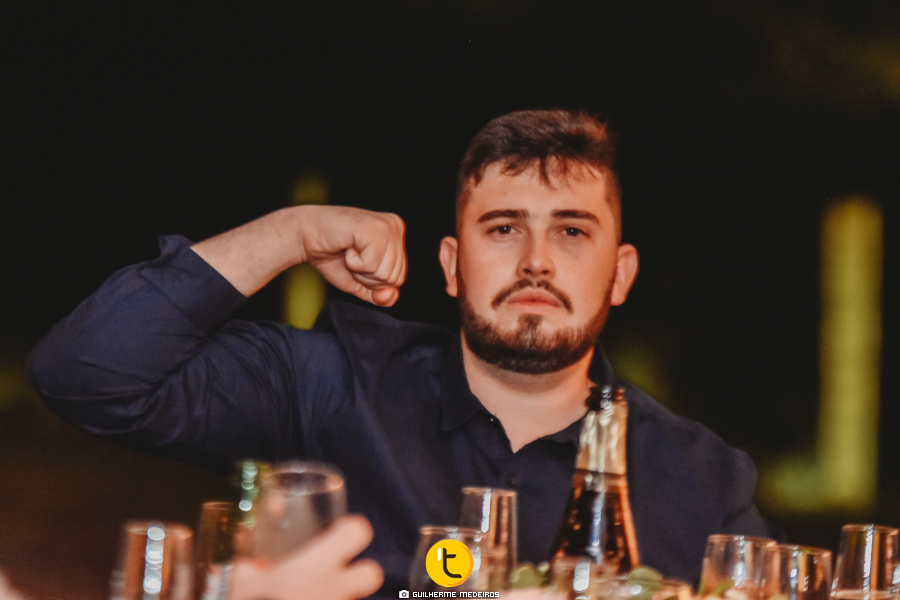In the photograph, a white man with short brown hair, a brown goatee, mustache, and beard, is facing the camera with a serious expression. He appears to be in his 20s or 30s and is wearing a dark blue button-down dress shirt with his right sleeve rolled up past the wrist. His right arm, though it appears on the left side of the image from our vantage point, is raised near his head in a bicep curl with his fist clenched, as if posing to show off his muscle. 

In front of him, there is an assortment of clear glasses and prominently, an amber-colored bottle with gold foil at the neck, suggesting it might be a bottle of wine or beer. The setting appears to be very dark, with a mostly black background accented by streaks of yellow-green light. Additionally, on the bottom left-hand side of the image, there's another person’s hand grasping a wine glass. The overall scene suggests a casual yet enigmatic moment captured in a dimly lit environment.